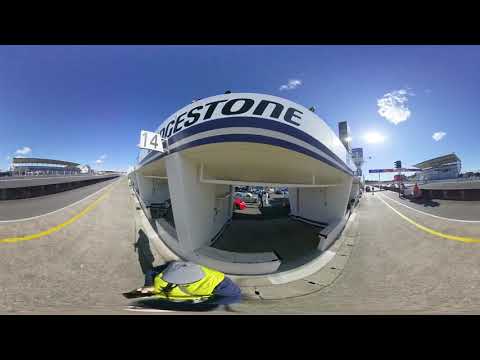This detailed image captures a panoramic, wide-angle view of a racetrack on a brilliantly clear, sunny day. Prominently featuring building number 14, the Bridgestone-branded structure is easily identified by its rounded top and garage entrance, which allows access to the track. In the foreground stands a yellow vehicle with a distinctive round cylinder on top and a pointed black nose, accompanied by a person dressed in black standing nearby. The spacious track itself extends into the distance, framed by stands on both the left and right sides. Further elements include white and yellow lines marking the track, a paddock area, and the finish line on the right. The sky overhead is pristine and blue, indicative of perfect weather conditions. Additionally, a man wearing a yellow jacket is also visible, contributing to the vivid scene typical of a bustling race day.